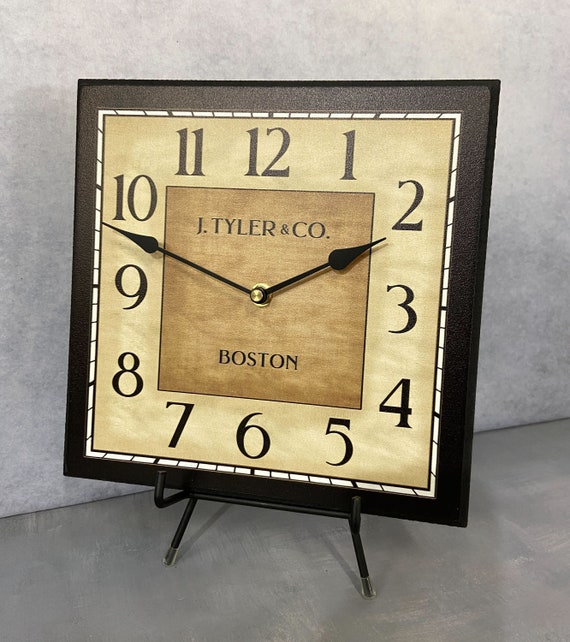The photograph features a vertically-oriented rectangular image of a distinctive square clock resting on a small black metal easel. The clock sits on a gray surface with a lighter gray wall in the background. The outer frame of the clock is dark, likely made of wood, with a decorative edge and thin white trim. The interior of the clock displays large black numbers from 1 to 12 against a light brown background, with a darker brown square at its center. Black hands, with rounded and pointed tips, indicate the time: the hour hand is at 2, and the minute hand is between 9 and 10. The inner dark brown square contains text at the top reading "J. Tyler & Co." and at the bottom, "Boston." The overall design is complemented by the black metal easel, which has curved hooks at the front and small legs peeking out beneath the clock.